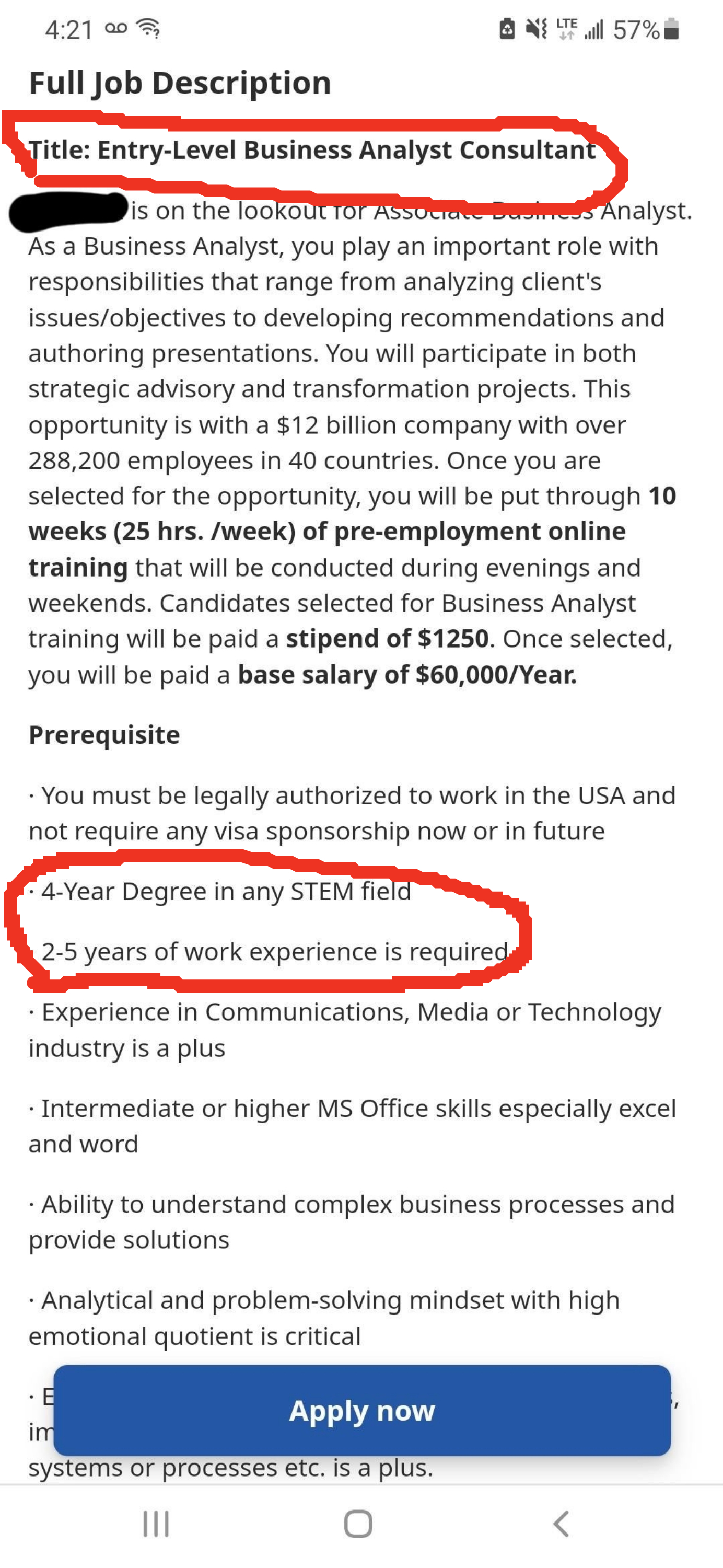**Caption:**

The image displays a job listing on a white background with detailed information about an entry-level business analyst consultant position. The title "Entry-Level Business Analyst Consultant" is prominently circled in red at the top of the listing, alongside a header that reads "421, 57% battery" and "Full Job Description."

The job description states that the first word is blacked out but indicates the company is seeking an associate business analyst. The role involves significant responsibilities that include analyzing client issues and objectives, developing recommendations, and creating presentations. Furthermore, the position entails participation in both strategic advisory and transformation projects.

The opportunity is with a prestigious company valued at $12 billion, boasting over 288,200 employees across 40 countries. Selected candidates will undergo 10 weeks of pre-employment online training, amounting to 25 hours a week, primarily conducted during evenings and weekends. A stipend of $1,250 will be provided for this training period. After training, the candidates will receive an annual base salary of $60,000.

Outlined in red, the prerequisites specify that candidates must be legally authorized to work in the USA without requiring visa sponsorship both currently and in the future. The preferred qualifications include a four-year degree in any STEM field and two to five years of relevant work experience, with experience in the communications, media, or technology industries considered a plus. Proficiency with MS Office tools, especially Excel and Word, is necessary, along with the ability to comprehend complex business processes and devise solutions. A strong analytical and problem-solving mindset accompanied by high emotional intelligence is essential for the role.

At the bottom of the listing, there is a prominent blue "Apply Now" button, followed by a navigation bar featuring three lines, a square icon, and a left arrow.